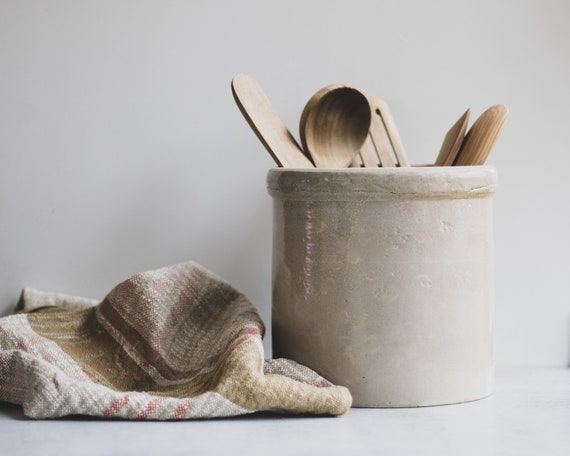In the image, a simple glazed ceramic vase resembling a coffee can sits prominently on a white countertop against a white wall. The vase, used as a utensil holder, contains several wooden kitchen utensils, including spatulas, spoons, and a scraper, some with visible handles and some partially obscured. To the left of the vase lies a rustic, patchwork-style dish towel, composed of various fabric pieces in plaid and gauzy patterns, evoking a linen-like, old, and worn appearance. The muted colors of the cloth vary from white to tan, with some light brown streaks. The overall setting conveys a minimalist and rustic aesthetic, with a cohesive white and gray color palette.